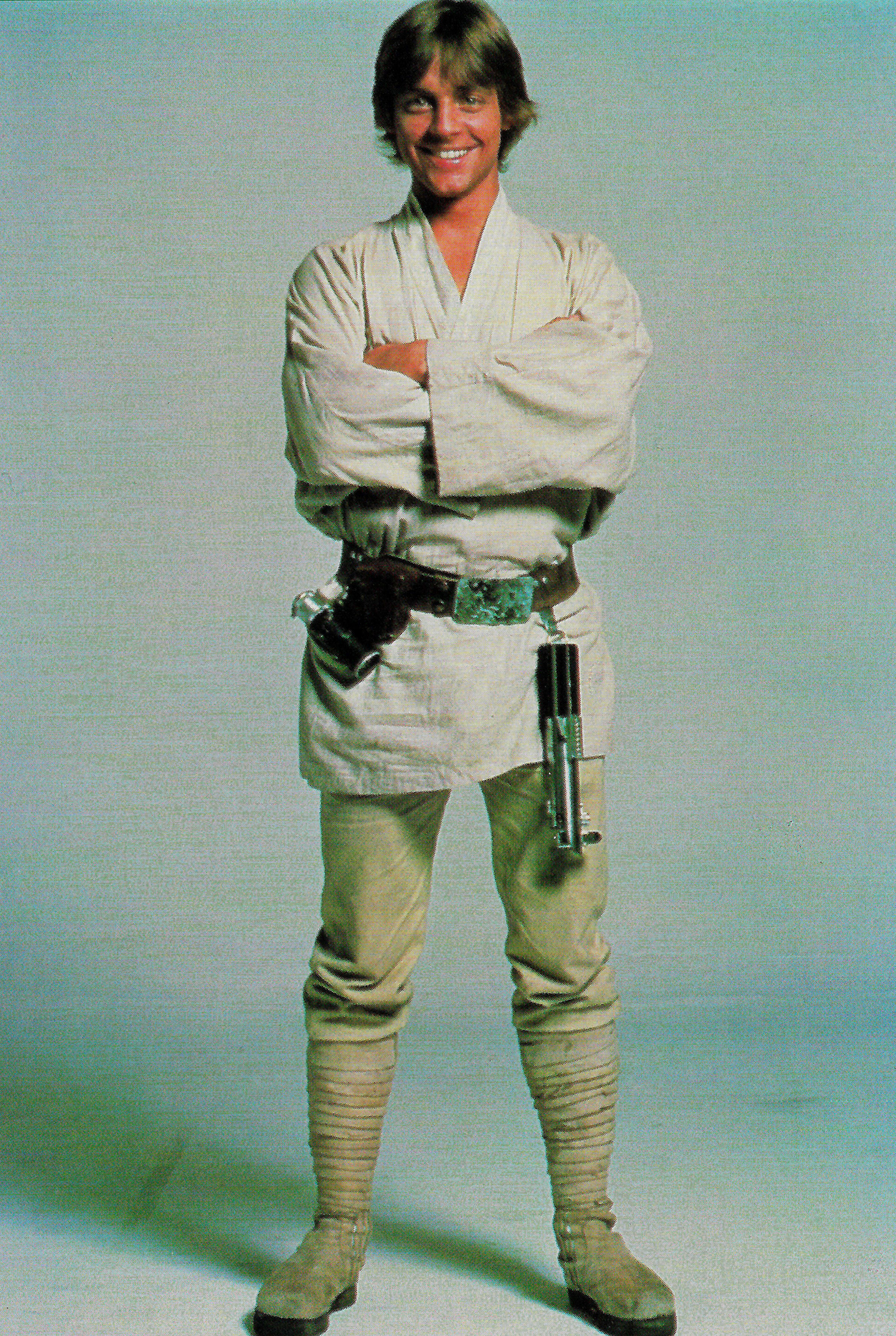The promotional photograph features Mark Hamill as Luke Skywalker from the original Star Wars trilogy, likely taken during the early '80s or possibly 1977. Dressed in an iconic Jedi outfit, Luke sports a white long-sleeve shirt forming a V-neck, off-white pants, and white boots. His costume is completed with a brown utility belt featuring a green buckle, a lightsaber, and various gadgets, possibly a flashlight and other tools. Luke stands against a white studio background, evoking a simple yet timeless aesthetic. With medium-length brown hair that touches his ears, he crosses his arms and offers a friendly, confident smile directly into the camera. The image captures a youthful and earnest portrayal of the character, exuding both charm and heroism.